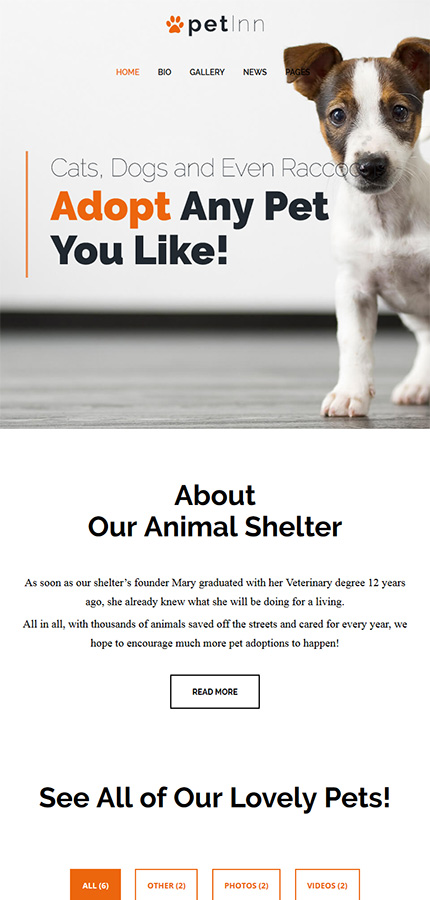A mobile phone screenshot showcasing a pet adoption app. At the top of the screen is an orange paw icon with the word "Pet" in bold black text and "in" in regular black text. Below the icon are navigation tabs: "Home" in orange, and "Bio," "Gallery," and "News" in black text. 

On the main screen, a puppy stands on a white floor background, positioned to the right of an orange vertical line. To the left of the line, the text reads: "Cats, dogs, and even raccoons. Adopt any pets you like." The phrase "Adopt any pets you like" is prominently displayed, with "Adopt" in orange and "any pets you like" in bold, dark text.

Centered underneath is a section titled "About our animal shelter" in black text, followed by several sentences in smaller black text. Below this text is a white rectangle with a black outline containing the words "READ MORE" in all caps. 

Further down, there's a message saying "See all of our lovely pets!" in black text. At the bottom of the screen, four buttons are outlined in orange: "All," "Other," "Photos," and "Videos," each with numbers in parentheses indicating the count of items available (e.g., All (6), Other (2), Photos (2), Videos (2)). The "All" button is selected, indicated by its orange shading, while the other buttons remain white with an orange outline.